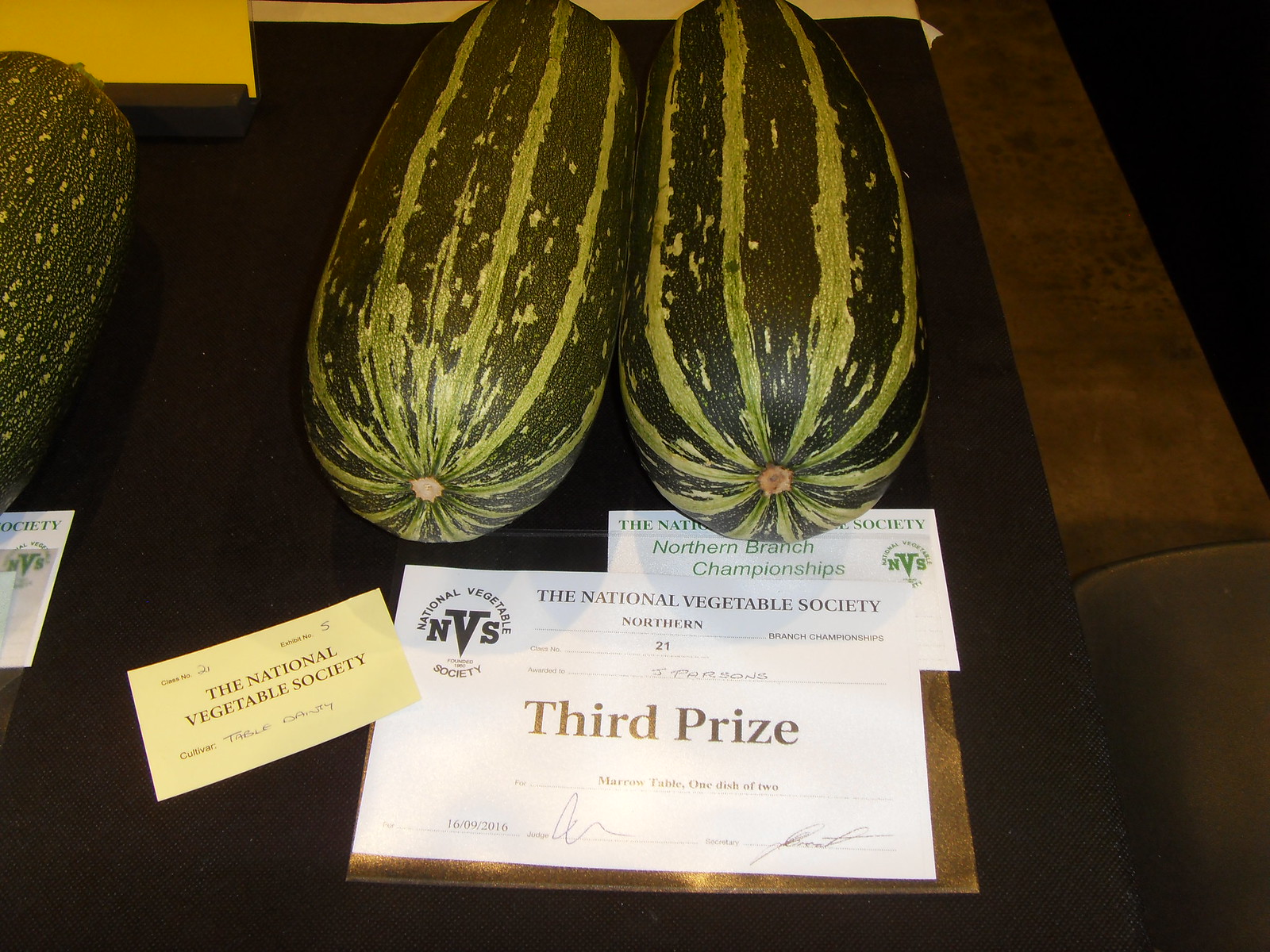In this image, two striped green watermelons rest side by side on a black table. Both melons exhibit a dark and light green striped pattern and are positioned with their ends facing the camera. Surrounding the melons are various documents related to their recognition in a vegetable growing competition. Prominently displayed is a card from the National Vegetable Society, accompanied by a certificate indicating a third prize win in a competition, likely within the squash category. The certificate features signatures and the name 'National Vegetable Society Northern Branch Championships.' Additionally, there's another squash in the upper left of the frame with an adjacent card, though the specifics of its recognition are not visible. This scene depicts the accolades granted in a prestigious vegetable competition.